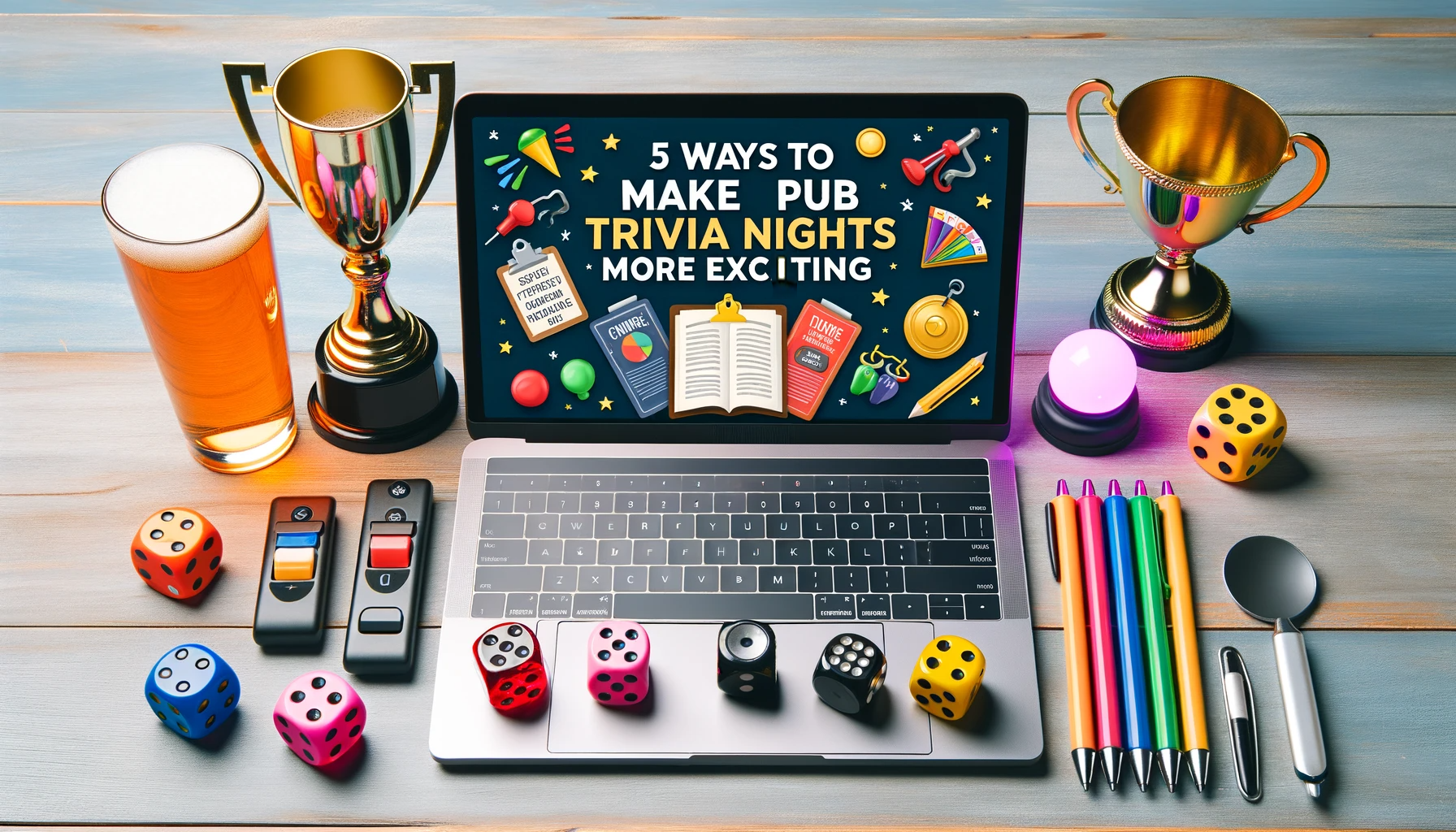This detailed digital artwork features an open laptop prominently displaying the text "Five Ways to Make Pub Trivia Nights More Exciting." Positioned on the keyboard’s trackpad are five colorful dice. Flanking the laptop screen on both sides are two gleaming gold trophies— the one on the left, taller with a slender design, stands beside a pint of beer emitting an unrealistic bright orange glow. Below these, two types of buzzers, likely for trivia games, and three additional dice are visible. On the right side of the laptop, another gold trophy, shorter and more stereotypically shaped, is present amidst a radiant purple orb casting a vivid magenta hue. Nearby, a set of five pens—two yellow, one green, one blue, and one pink—are scattered around, along with a marker-like item and what appears to be a small scoop. This array of objects, along with the vibrant and somewhat inconsistent lighting effects, suggests the image might be AI-generated.